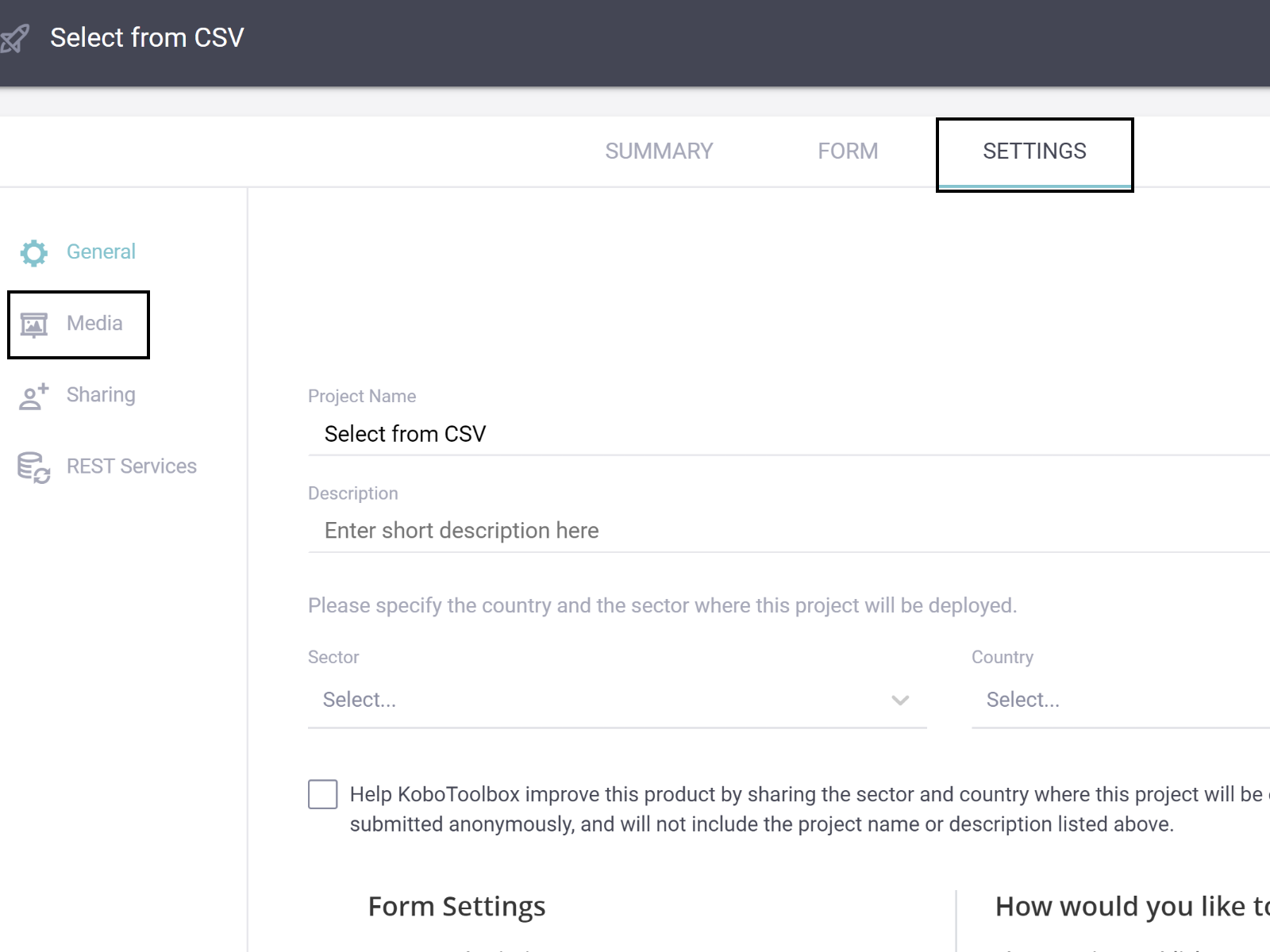**Caption:**

This screenshot displays a user interface from a website or application featuring a black and white input selection field with a touch of blue text. At the top, a gray background stripe houses the text "Select from CSV," with a gray rocket ship icon and light lines beside it. Below this, there are three tabs: Summary, Forms, and Settings, with the Settings tab currently outlined in black and selected. Below the tabs, a vertical menu on the left highlights several options including "General" (with a gear icon in blue), "Media," "Sharing," and "REST Services," all outlined in black.

On the right panel, multiple fields are visible:
- "Project Name" with an input field to select from a CSV.
- "Description" with a placeholder text for entering a short description.
- A prompt to specify the country and sector for project deployment with corresponding drop-down menus for "Sector" and "Country."
- An unchecked checkbox option urging users to help improve the Kobol Toolbox product by sharing deployment details about the sector and country, though the full text is partially cut off on the right side.

Below these fields, there is a section titled "Form Settings" with text to the right that is partially obscured and thus cannot be fully detailed.